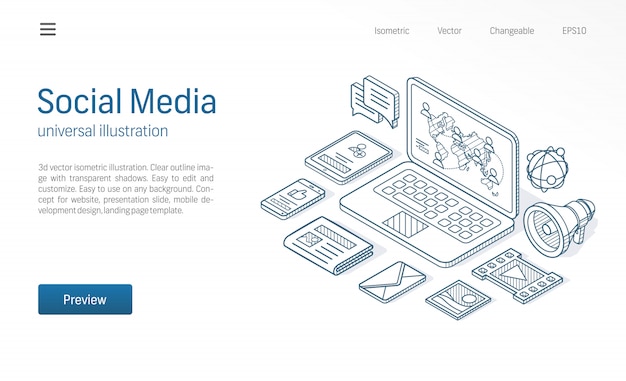The infographic features a detailed 3D vector isometric illustration with a blue and white color scheme, combining a variety of social media and communication-related elements. The primary focus of the image is a central laptop surrounded by various icons: a megaphone in the back right corner, speech bubbles on the left, an envelope and newspaper positioned in front, along with additional icons including a phone, a tablet, a video symbol, and an image symbol. Notably, a network symbol comprising a ball with surrounding balls and lines is also present. The text overlays describe the graphic as a "Social Media Universal Illustration, 3D Vector Isometric Illustration" with attributes like "Clear Outline Image with Transparent Shadows," specifying that it is "Easy to Edit and Customize" and "Easy to Use on Any Background." The design, intended for use as a website or landing page template, offers concepts for presentation slides, mobile development, and more. Additionally, a prominent blue "Preview" button suggests interactivity, with technical details mentioning "Isometric, Vector, Changeable, EPS10." The cohesive blue and white design elements provide a clean and modern look suitable for various digital applications.